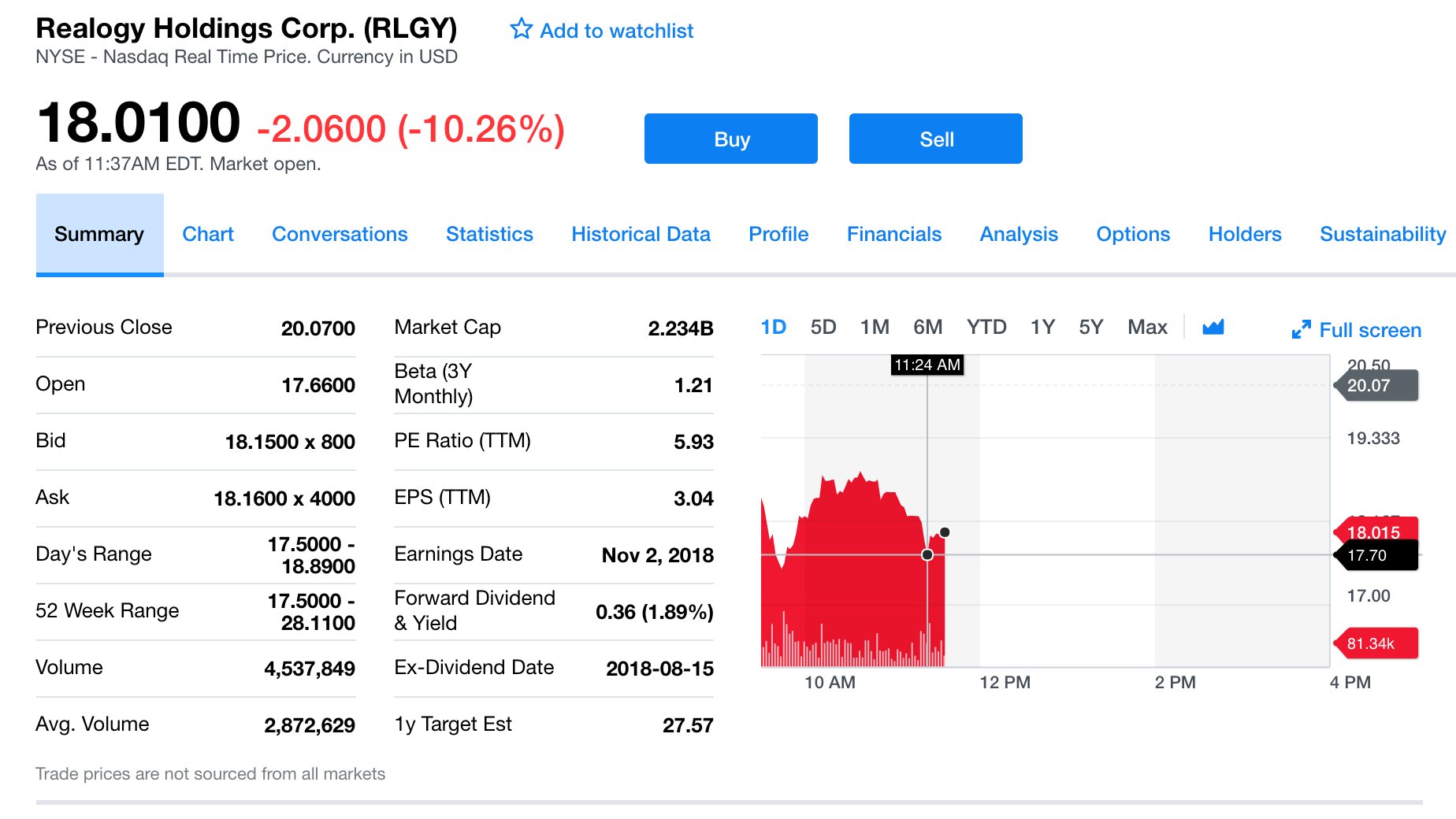In the top left corner of the image, the name "Realology Holdings Corp. (RLGY)" is displayed prominently. To the right of this, there is an unfilled blue star icon accompanied by the text "Add to Watchlist" in blue. Just below the stock name, it reads "NYSE - NASDAQ Real-Time Price. Currency in USD."

The current stock price is shown as $18.0100, with a notable decline of -$2.0600, or -10.26%, indicated right next to it in parentheses. Adjacent to these figures, there are two rectangular buttons labeled "Buy" on the left and "Sell" on the right.

Towards the lower left section of the image, there is a navigation menu with various sections listed: "Summary" (highlighted with a blue underline and light blue background), "Chart", "Conversations", "Statistics", "Historical Data", "Profile", "Financials", "Analysis", "Options", "Holders", and "Sustainability".